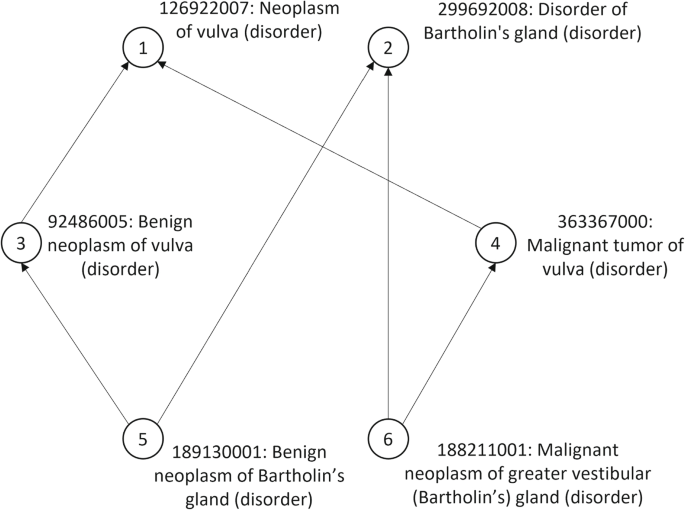The image is a black-and-white medical diagram that appears to come from a scientific textbook. It consists of six numbered data points, each labeled with specific medical conditions and numerical codes that likely correspond to medical classification systems. The diagram includes various lines connecting these points, indicating relationships between them. The specifics are as follows:

1. **Neoplasm of Vulva Disorder** (Code: 126922007)
2. **Disorder of Bartholin's Gland** (Code: 299692008)
3. **Benign Neoplasm of Vulva** (Code: 92486005)
4. **Malignant Tumor of Vulva** (Code: 36336700)
5. **Benign Neoplasm of Bartholin's Gland** (Code: 189130001)
6. **Malignant Neoplasm of Greater Vestibular Bartholin's Gland** (Code: 188211001).

Each condition is connected through lines that illustrate the potential progression or relationship between various neoplasms and disorders of the vulva and Bartholin's gland. This diagram likely serves as an educational tool for understanding the links between different vulvar and Bartholin's gland disorders, potentially related to oncological studies or gynecological health.